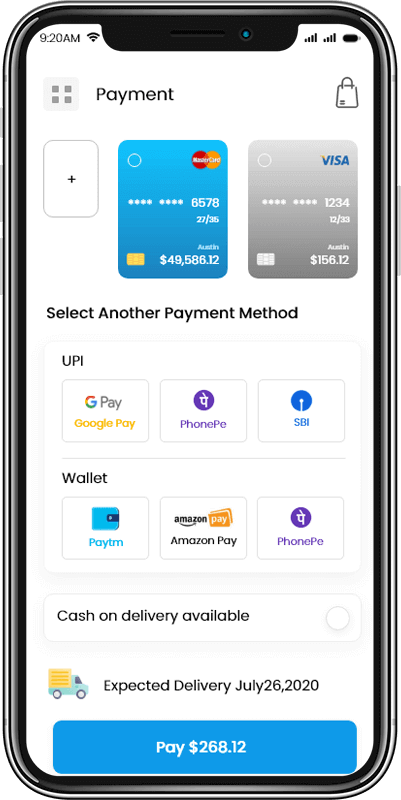The image displays a mobile phone screen showing an online payment interface. The phone has silver edges and a black-tipped top. At the top of the screen, the status bar indicates a 920m 4G connection with full signal strength and a fully-charged battery.

The main section of the screen features various payment options. A shopping bag icon is visible, and the top payment method displayed is MasterCard, rated with four stars. The associated details include two sets of numbers: 6578 and $49,586. Below that, a Visa card is shown, also rated with four stars, listing numbers 1234 and $156. 

Additional payment methods include UPI, Google Pay, PhonePe, and SBI. There's a wallet option labeled "Pay ATM," as well as Amazon Pay and PhonePe. The interface also allows for cash on delivery. A truck icon indicates an expected delivery date of July 26, 2020. 

At the bottom portion of the screen, a blue rectangle button is labeled "Pay $268.12." The edges of the screen are grey, and various buttons are also visible.